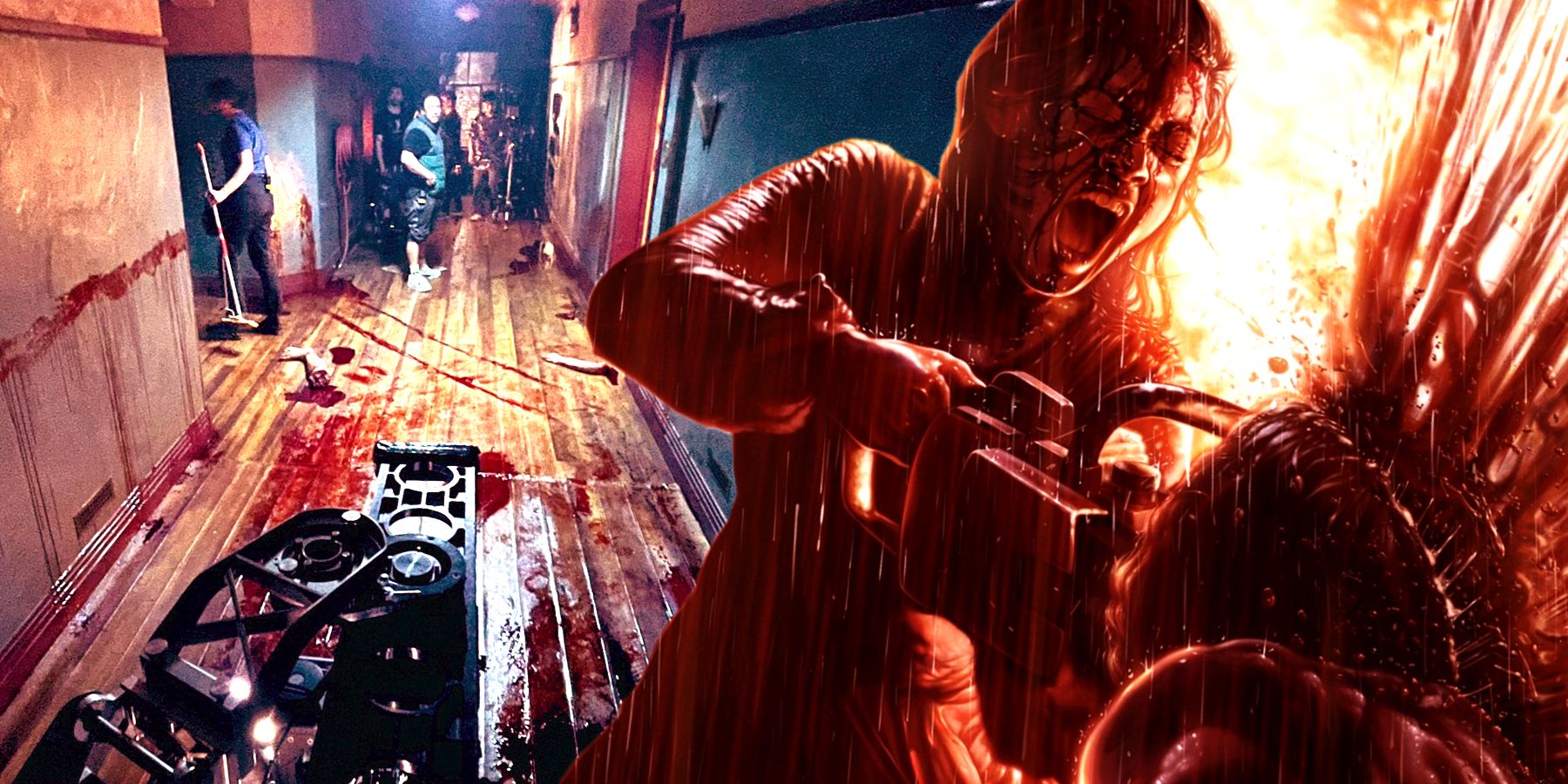The image depicts a dramatic scene on what appears to be a movie set, likely from a horror film. Dominating the right side of the image is a blood-soaked individual, presumably an actress, wielding a chainsaw and screaming, her face covered in fake blood. She seems to be sawing into something that resembles a giant, grotesque plant, reminiscent of a mutated Venus flytrap, with splatters of red indicated to be blood spraying outward.

The setting is a dimly lit, wooden hallway that is stained with blood. On the left side of the image, a group of observers, likely the film's crew, watch casually. Among them is a man holding a broom, walking away. Visible on the hardwood floor is a black mechanical device that looks like it could be used to hold a camera, reinforcing the idea of a controlled film set.

The composition highlights the contrast between the violent, chaotic scene of the actress and chainsaw on the right, and the calm, nonchalant demeanor of the crew on the left. This juxtaposition, along with the presence of filmmaking equipment, underscores the artificiality of the horror, emphasizing its nature as a staged movie production.